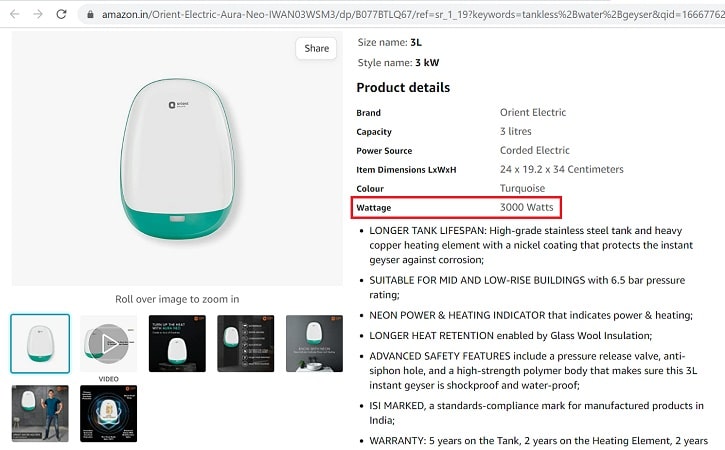This is a screenshot of an Amazon India product page. The URL at the top begins with "Amazon.in." On the left side of the page, there are product images, with the largest being an egg-shaped device that is predominantly white with a teal bottom and a slim teal outline. Below this main image, there are seven thumbnail images, and the main picture is circled in green.

On the right side, there is a table detailing the product's specifications, including the brand, capacity, power source, item dimensions, color, and wattage. The wattage is specifically highlighted with a red outline. Below this table, there appears to be a green screen bar prominently displayed, followed by text that reads "bottom forefront" and "top front 27 time screen." This section seems to showcase the monitor's capabilities in displaying all of the device's waterproof components. The page also includes additional information and shared links relevant to the product.